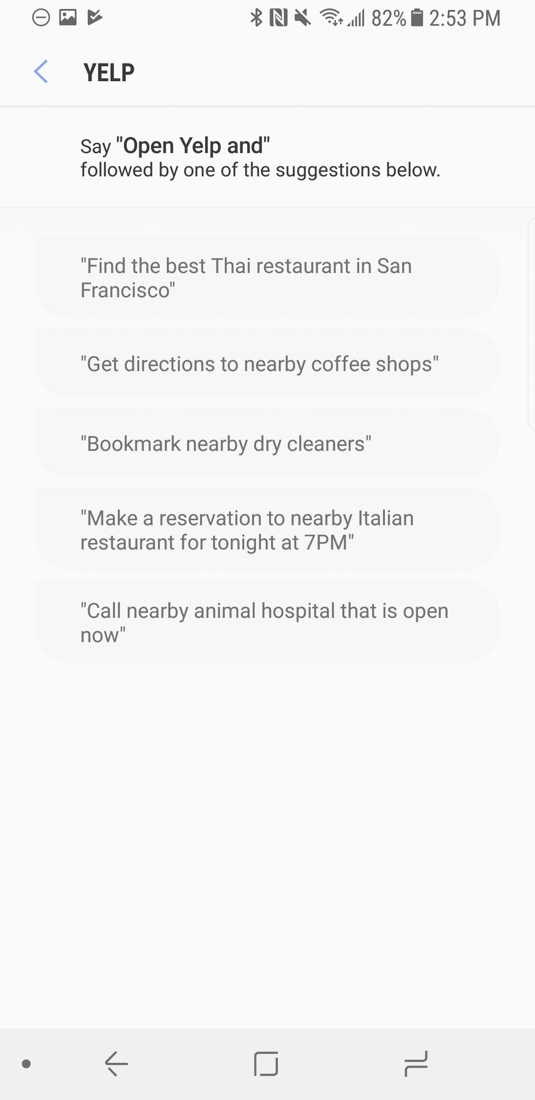A screenshot of an Android device at 2:53 PM with 82% battery remaining. At the top of the screen, "YELP" is displayed in bold letters. Below that, a prompt reads, "Say 'Open YELP'" in bold, followed by the instruction to "use one of the suggestions below." Five suggestions are listed:

1. "Find the best Thai restaurant in San Francisco."
2. "Get directions to nearby coffee shops."
3. "Bookmark nearby dry cleaners."
4. "Make a reservation at a nearby Italian restaurant for dinner tonight at 7 PM."
5. "Call a nearby animal hospital that is open now."

The image highlights various voice commands that can be used with the YELP app, showcasing its versatility and convenience.